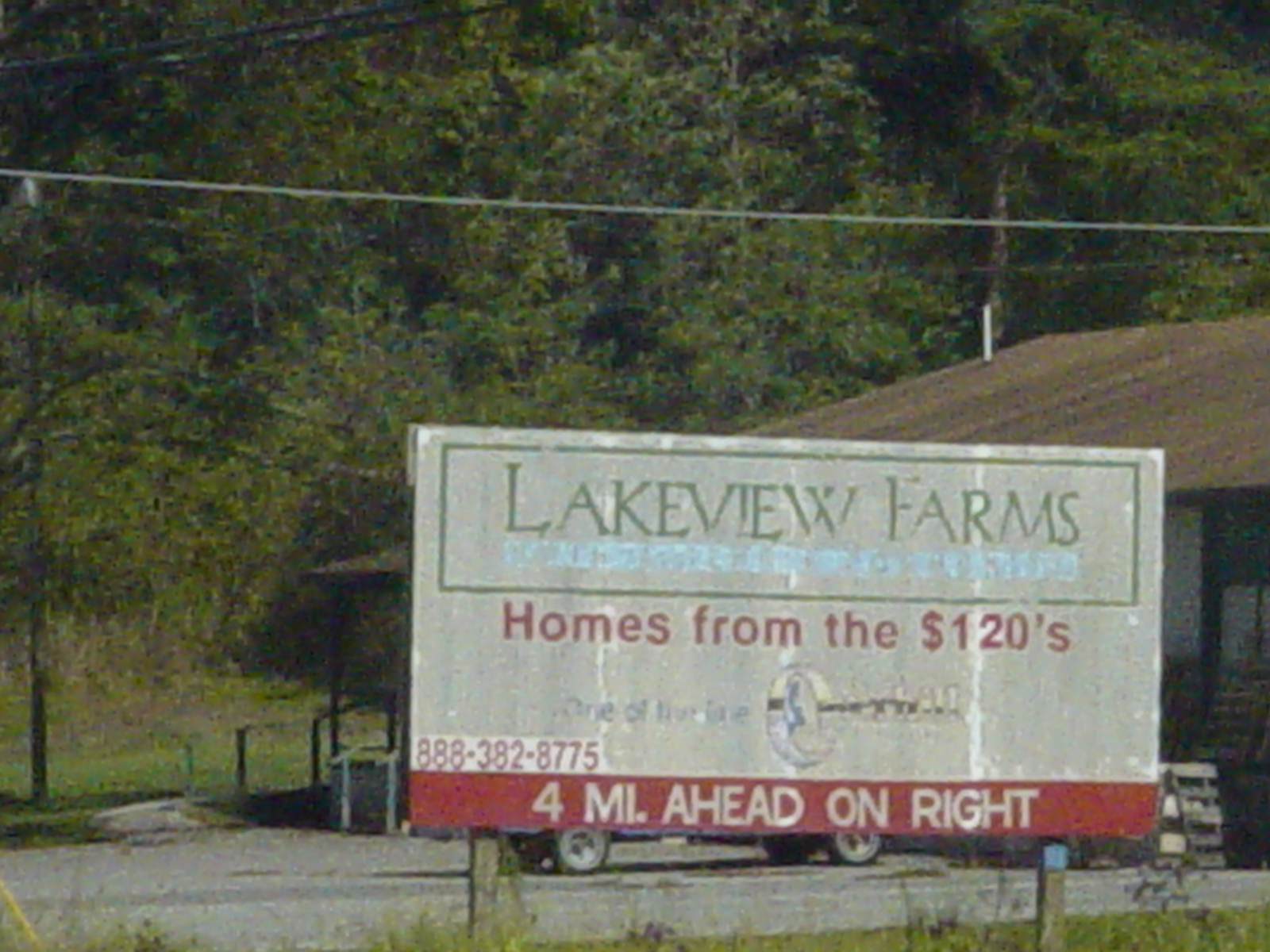The image features a faded, grainy photo of a billboard for Lakeview Farms, advertising homes starting from the $120s. The sign, which is somewhat old and worn, stands in the bottom right-hand corner of the picture and is framed by wooden fence posts. It includes a prominent red banner at the bottom that reads, "Four miles ahead on the right," along with a contact number: 888-382-8775.

Behind the sign stands an indistinct building structure with only the roof visible, suggesting it might be an office or some type of facility. A car appears to be parked nearby, indicated by visible tires beneath the sign. The area around the sign is rather overgrown with long, unmowed grass.

Further in the background, a dense forest of tall, green trees extends up a mountain face, giving the impression that the location is nestled between a highway and a forested area. The scene is calm and appears to be quite rural, with no noticeable traffic and the surroundings contributing to an isolated, serene environment.